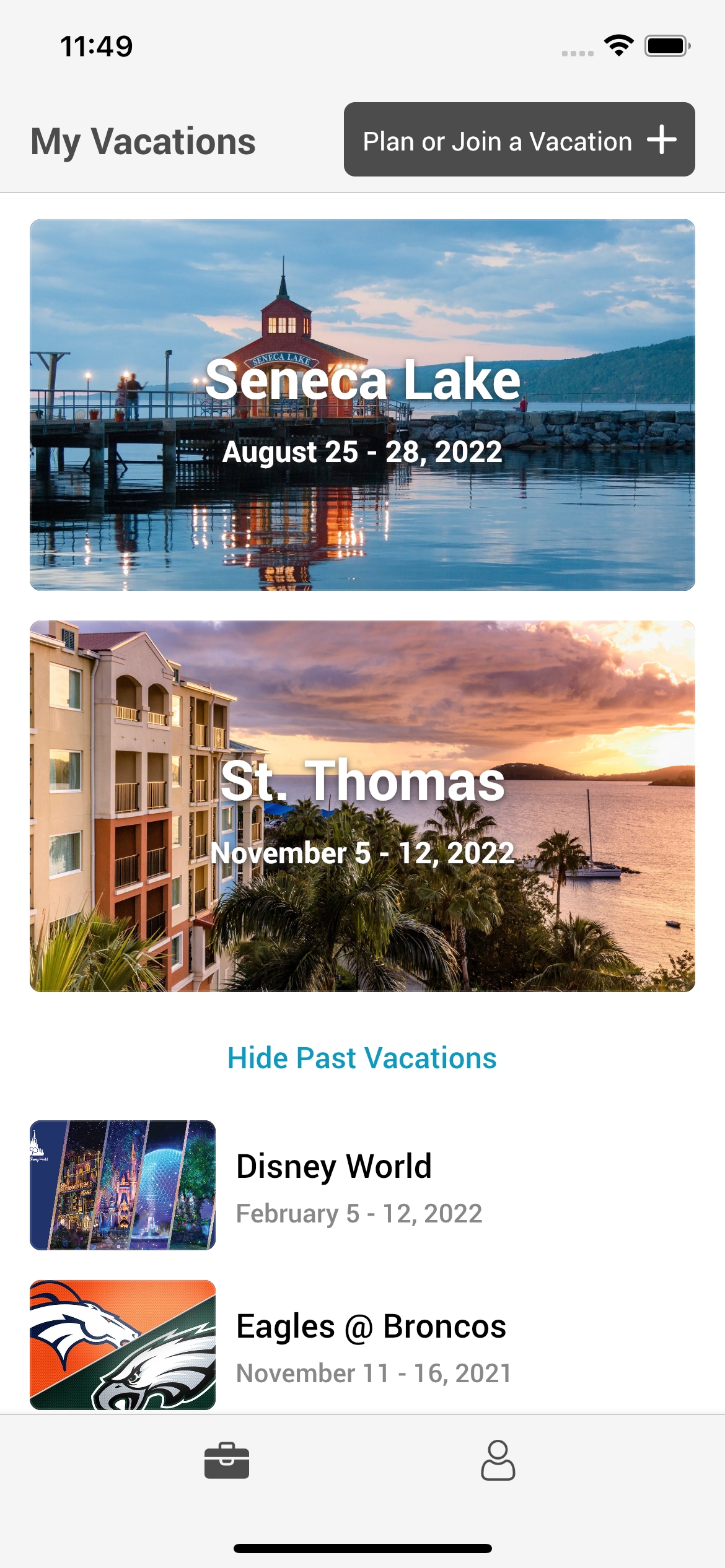The image showcases a travel app interface with multiple sections. At the very top, the screen displays the time, a WiFi symbol, and battery percentage. Grey text reads "My Vacations," with a subtitle prompting users to "Plan or join a vacation." Adjacent to this text is a grey button marked with a plus sign.

Below, the app lists an upcoming vacation titled "Seneca Lake, August 25-28, 2022," accompanied by an image featuring tranquil water, a boardwalk, surrounding rocks, and distant mountains. Beneath that, there's another planned vacation to "St. Thomas, November 5-12, 2022," represented by an image of a beachfront building by the waterfront.

A blue button labeled "Hide Past Vacations" allows users to manage their view of previous trips. Two past vacations are listed: "Disney World, February 5-12, 2022," featuring an image of a theme park, and "Eagles at Broncos, November 11-16, 2021," accompanied by logos of the Denver Broncos and Philadelphia Eagles football teams.

Near the bottom of the screen is a suitcase icon and the outline of a person's upper body, likely shortcuts to access the luggage and profile pages respectively. The background of the app is predominantly light grey and white, with various text elements enhancing the content.